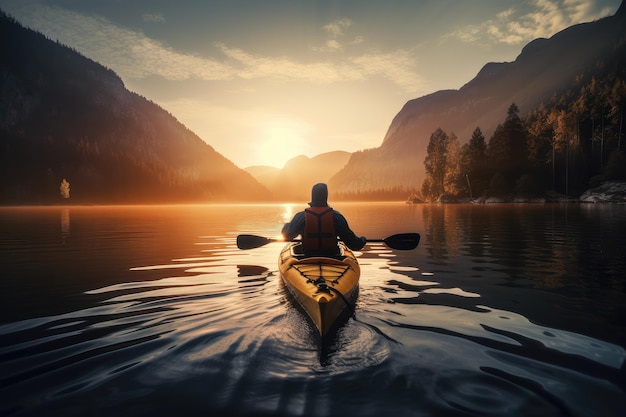The image depicts a serene outdoor scene featuring a lone kayaker, framed in a 3D-style, photographic graphic. The person, seen from behind with their back turned to the camera, is paddling a yellow kayak adorned with webbing in the back, wearing a red vest, and holding a double-paddle oar. They navigate through the calm waters of a large lake, creating gentle ripples. It's either sunrise or sunset, with the sun peeking vibrantly between a valley of two mountains. The sky above is a vivid blue, streaked with white clouds. To the right of the image, a dense cluster of green trees lines the shore, adding to the natural beauty and tranquility. The peaceful demeanor of the kayaker, gliding smoothly over the water, suggests a moment of solitary reflection and harmony with nature. The backdrop showcases the surrounding mountains, with distinct profiles: one on the left with a steady incline and the one on the right featuring a more jagged, zig-zagging silhouette, amplifying the scenic splendor of the setting.